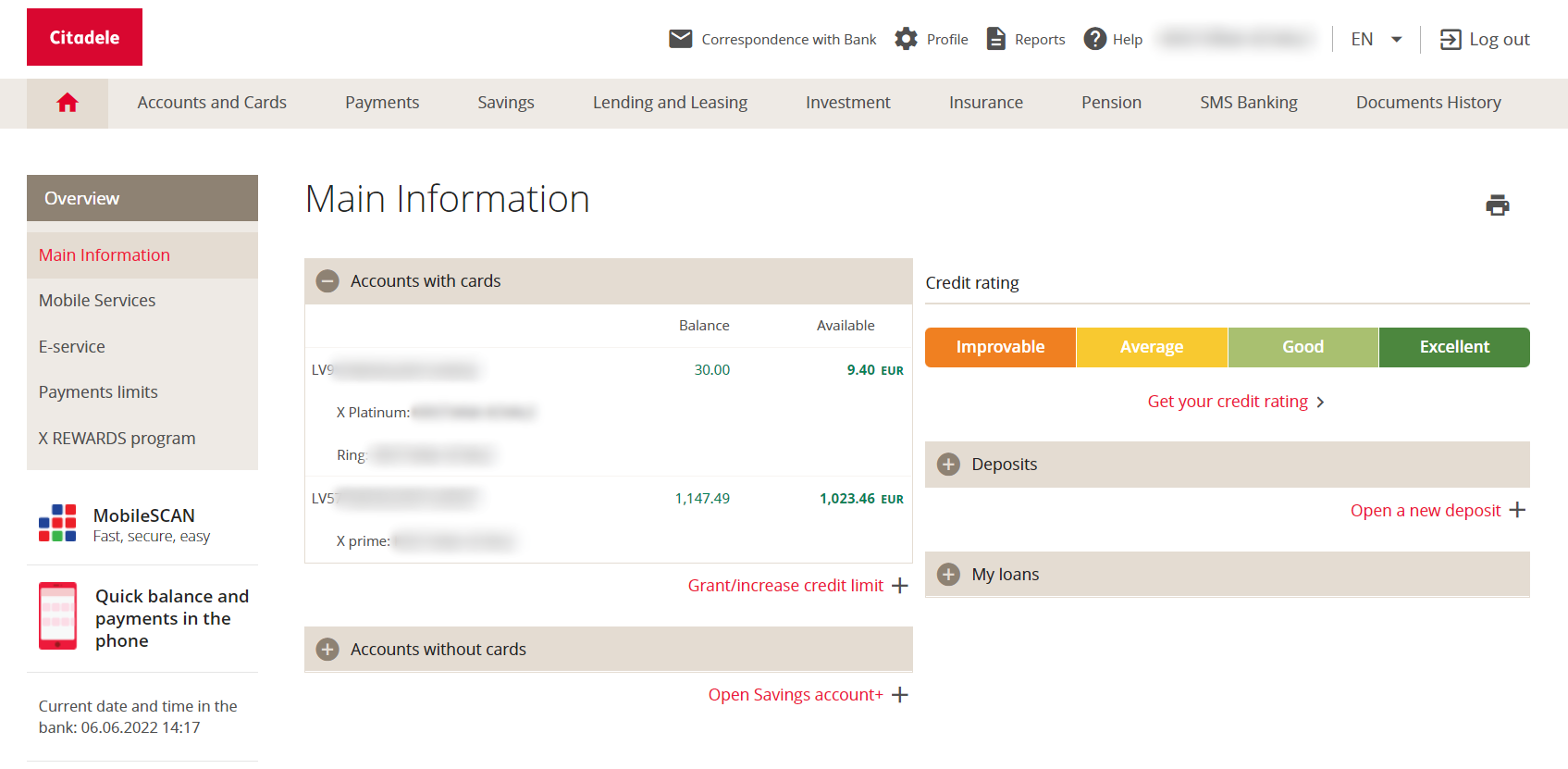The website interface of Citadel is detailed above. The Citadel logo, written in white text, prominently features in the top left-hand corner on a red button. Adjacent icons include:

- A coin symbol
- A mail icon
- Several navigation categories like correspondence with the bank, each highlighted as follows:
  - Settings icon labeled "Profile"
  - Reports icon labeled "Reports"
  - A help icon represented with a question mark in a circle

A redacted area, likely indicating the user's profile, is visible. Additional navigation features include a language option set to English and a logout button represented by an arrow within a box.

Below the primary navigation, there is a comprehensive menu bar listing several categories, each as a distinct title:

- Home (indicated by a red home icon)
- Accounts and Cards
- Payments
- Savings
- Lending and Leasing
- Investment
- Insurance
- Pension
- SMS Banking
- Documents History

Underneath these categories, the first row presents specific options such as:

- Overview
- Main Information
- Mobile Services
- E-Service
- Payments
- Limits
- X Rewards Program

The subsequent row includes segments like "Main Information" and "Credit Rating," arranged sequentially.

Overall, this layout offers a detailed and structured navigation system for users to manage various aspects of their banking and financial tasks.